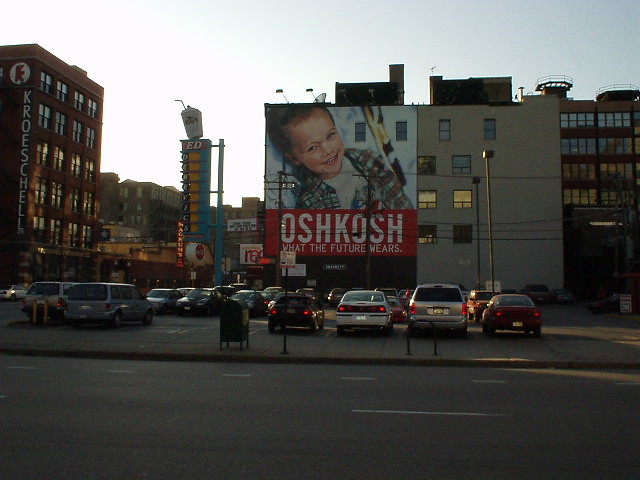The image features a vibrant scene with a prominent Oshkosh B'gosh poster in the background, emblazoned with the slogan "Oshkosh: What the Future Wears." In the foreground, a child is modeling a stylish jacket paired with a white shirt. A tall, white tower resembling a billboard looms in the background, adding a modern touch to the urban landscape. 

In the lower part of the image, a parking lot stretches out, leading to a quaint diner situated towards the back left. The diner's sign is a striking blue and prominently features a depiction of a milkshake complete with a straw and cherry on top, evoking a sense of nostalgic charm. 

On the right side, a series of apartment buildings rise up, suggesting a residential area. To the left at the top of the image, another building can be seen. The entire scene is anchored by a road running along the bottom of the image, tying together the bustling, multifaceted environment.